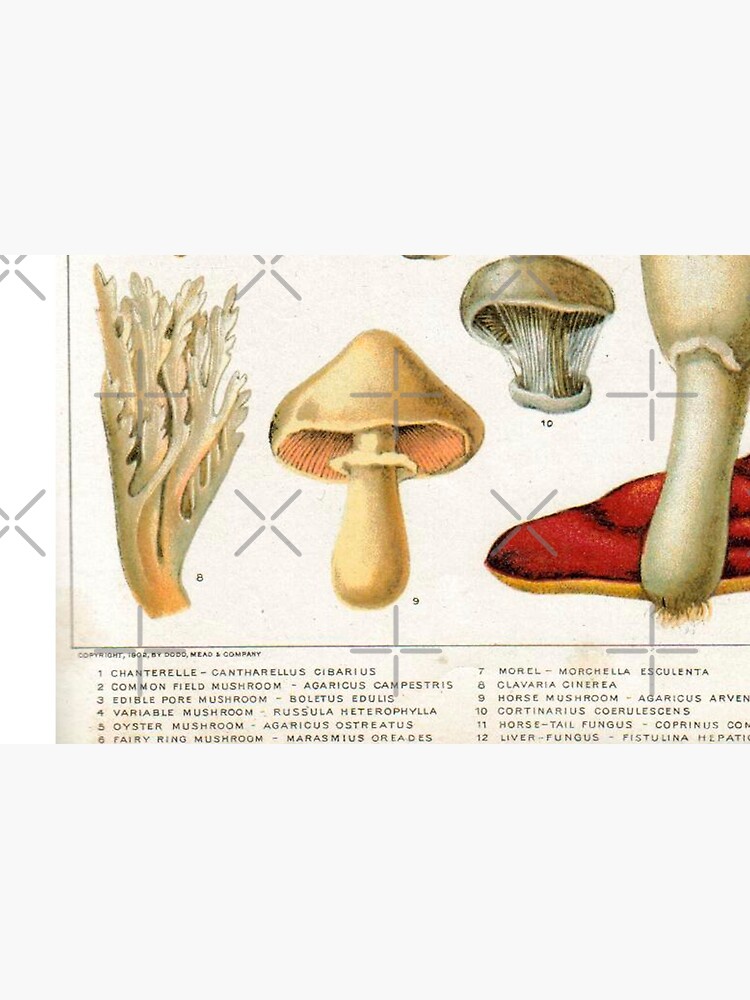This detailed image appears to be a page from an encyclopedia or textbook about mushrooms, set against a white background. The central focus is on four different types of mushrooms, each distinctly illustrated and numbered. 

To the far left is a mushroom resembling a piece of seaweed, numbered 8, characterized by its unusual slim and elongated structure. Next to it, numbered 9, is a more traditional-looking mushroom with a yellowish cap and stem. The third mushroom, numbered 10, is a grayish-brown mushroom similar in shape to the yellow one, but with noticeable filaments extending from its stem.

To the right of these is a mushroom stem without a traditional cap, seemingly just a stalk, and behind it lies a peculiar red, flat object that looks like a rock. Below this illustration is an array of scientific names and descriptions of various mushrooms, ranging from chanterelle to common field mushroom and others up to number 12. The writing is in block print but is too small to read clearly. This comprehensive illustration closely resembles educational material designed to provide detailed information about different mushroom species.